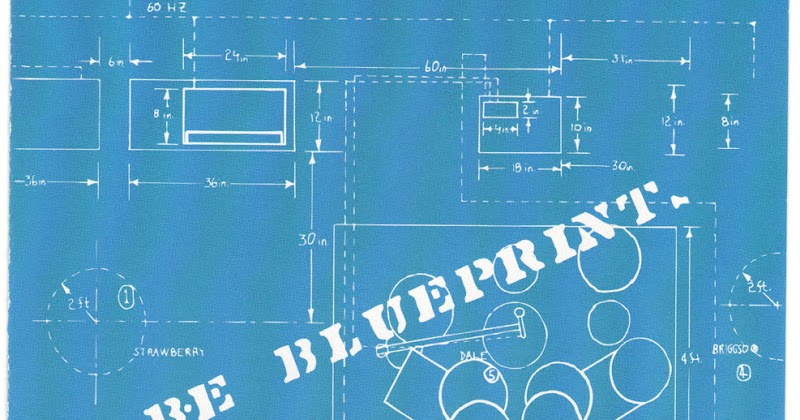The image is a detailed blueprint displayed on a blue background. Across the top, the bold, all-capitalized word "BLUEPRINT" is prominently featured in a block-style stencil form of lettering. From the bottom left to the top right corner, another word, partially cut off, angles diagonally upward.

In the top left corner of the blueprint, there is a large rectangle measuring 20 inches by 8 inches with a smaller rectangle at its bottom. Adjacent to the southwest of this rectangle is a circle with a radius of 2 feet, labeled "Strawberry," featuring clock hands and outlined in a dotted pattern.

To the right of the larger rectangle is another rectangle measuring 10 inches by 8 inches. Inside this rectangle, at the top left, is an even smaller rectangle measuring 2 inches by 4 inches. Below this smaller rectangle are numerous circles, some resembling pulleys, contained within a rectangular area measuring 4 feet by 8 feet. These circles fall under the label "blue-pinch."

At the bottom center of the blueprint, six circles are outlined in white. Additionally, three vertical circles are encased within a square outline along the side. Towards the right of these elements is another dotted circle with clock hands. Dotted lines run across the top, interspersed with multiple solid rectangles and squares, contributing to the intricate design layout of the blueprint.